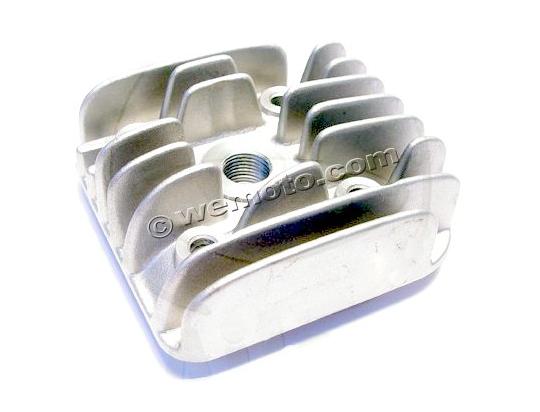The image features a metallic heat sink with a silvery-gold or chrome appearance. It consists of nine rows of metal fins running horizontally across a flat, rectangular tray-like structure. Each fin is designed to provide cooling functionality, typically used in vehicles or machinery. In the center of the heat sink is a prominent threaded screw hole, surrounded by a square pattern of four additional threaded screw holes located near the edges. These holes are positioned one per corner and are intended for securing the heat sink in place. The fins are arranged with two located at the top, one at the bottom, and additional full-length fins spanning the middle section, surrounding the large central screw hole. The metal surface is marked with a watermark reading "copyright weimoto.com," indicating the manufacturer's branding. The overall design appears robust, hinting at its potential applications in mechanical or industrial settings.